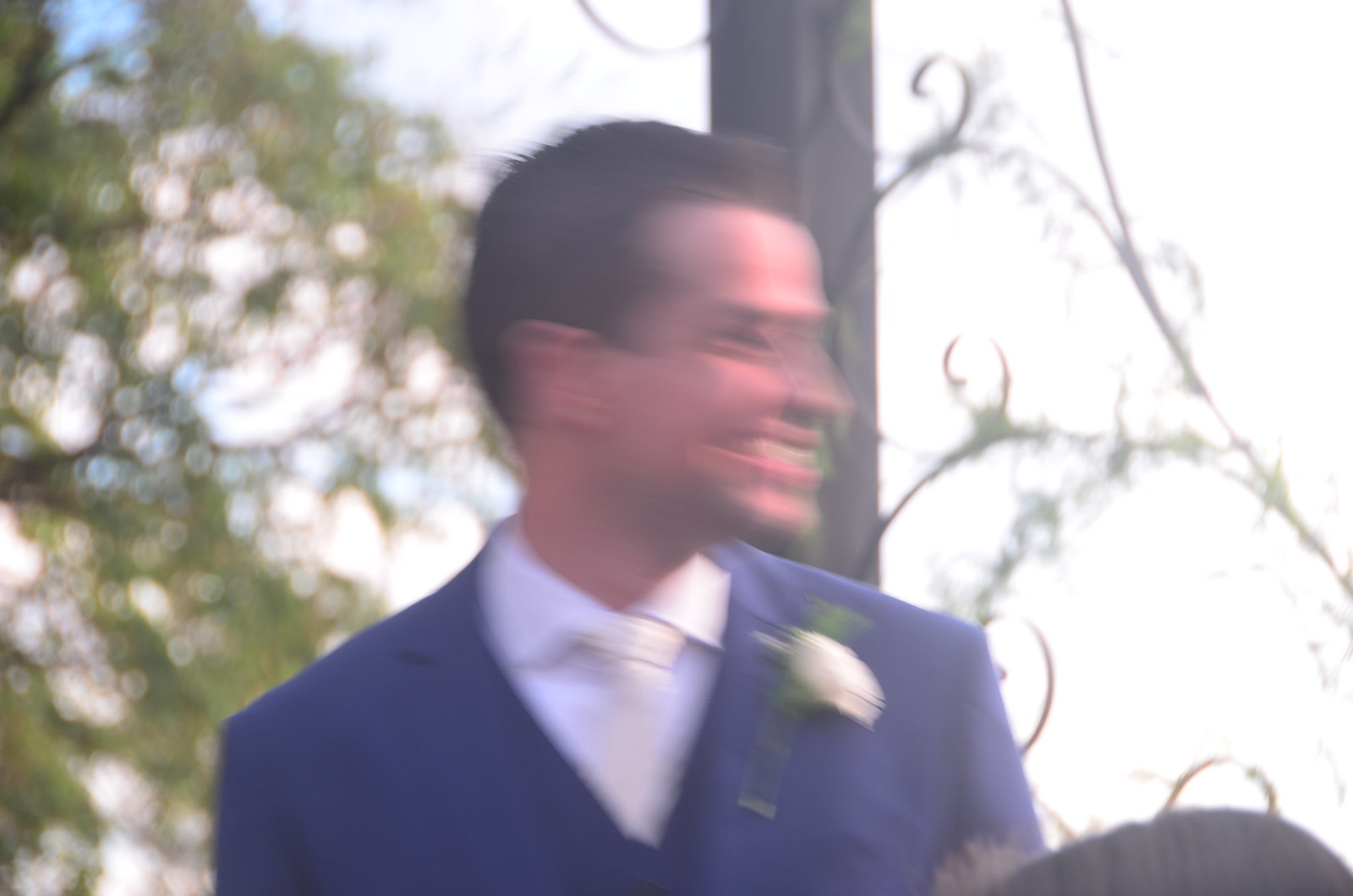This close-up, albeit very blurry, photograph captures a joyful man at what appears to be a wedding. He dons a tailored dark blue suit with a white shirt and an eggshell-colored tie, accentuated by a white flower pinned to his left lapel. His well-groomed dark brown hair is slicked back, and his dark eyes gleam as he smiles broadly, revealing his front teeth. The background includes a dappled light filtering through trees, a wooden post, and some metal wrought iron artwork, adding to the celebratory outdoor setting. The man’s head is turned at a 90-degree angle to the left, which might explain the motion blur, contributing to the overall liveliness of the image.